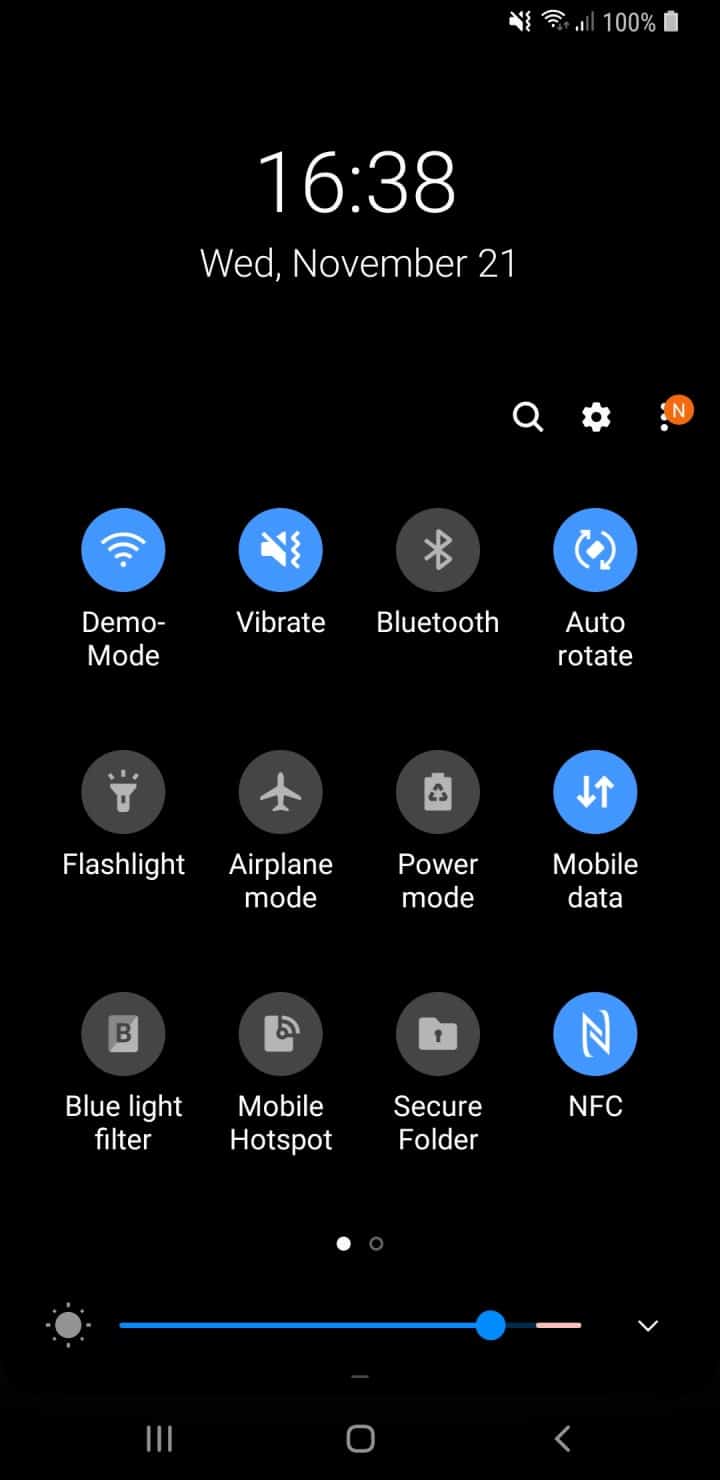This screenshot captures the main interface of a smartphone. At the top right corner, standard status icons are visible, indicating full battery at 100% and internet connectivity. The black background prominently displays the current time, 16:38, and the date, Wednesday, November 21st.

The main area consists of 12 circular icons, each representing different settings:

1. **Demo Mode (Highlighted in Blue)**: Active state, indicated by a blue circle.
2. **Vibrate (Highlighted in Blue)**: Currently active.
3. **Bluetooth (Gray)**: Not active.
4. **Auto Rotate (Highlighted in Blue)**: Active.
5. **Flashlight (Gray)**: Not active.
6. **Airplane Mode (Gray)**: Not active.
7. **Power Mode (Gray)**: Not active.
8. **Mobile Data (Highlighted in Blue)**: Active with two arrows.
9. **Blue Light Filter (Gray)**: Not active.
10. **Mobile Hotspot (Gray)**: Not active.
11. **Secure Folder (Gray)**: Not active.
12. **NFC (Highlighted in Blue)**: Active.

At the bottom, navigation indicators show two dots, with the first dot filled in white, indicating that we are on the first page of the settings menu. Beneath this, a status bar with a blue progress line and a circular sunburst icon on the left side, along with a downward-pointing caret on the right, is visible, likely representing brightness or volume control.